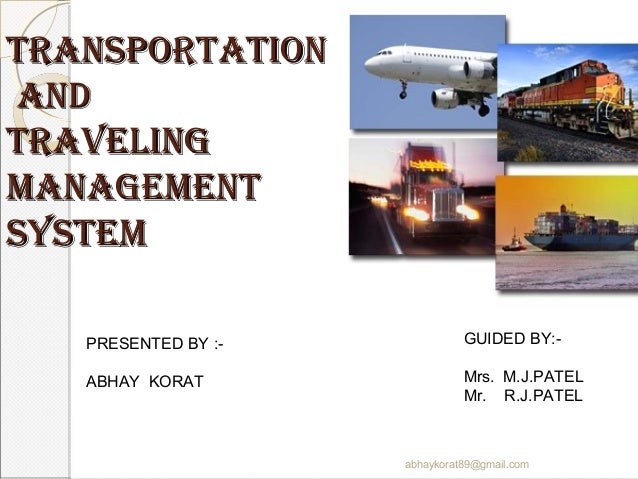The image appears to be an advertisement, potentially for a transportation or logistics management system. The layout is a large white square with a light gray vertical strip running down the left-hand side. Within this strip, the title "Transportation and Traveling Management System" is prominently displayed in dark brown text. Underneath this header, in smaller black text, it says "Presented by Abhay Kaurat." Further below, the text reads "Guided by Mrs. M. J. Patel and Mr. R. J. Patel."

The right side of the advertisement features a collage of four images. The top left image is a white passenger jet soaring through a clear blue sky. Below this is a red semi-truck traveling on a highway. Adjacent to the airplane is a red and yellow train engine, also in a sunny, clear sky setting. Underneath the train, there is a barge on the ocean with a beautiful sunset in the background. At the bottom of the image, in gray text, the email address "AbhayKaurat89@gmail.com" is provided.